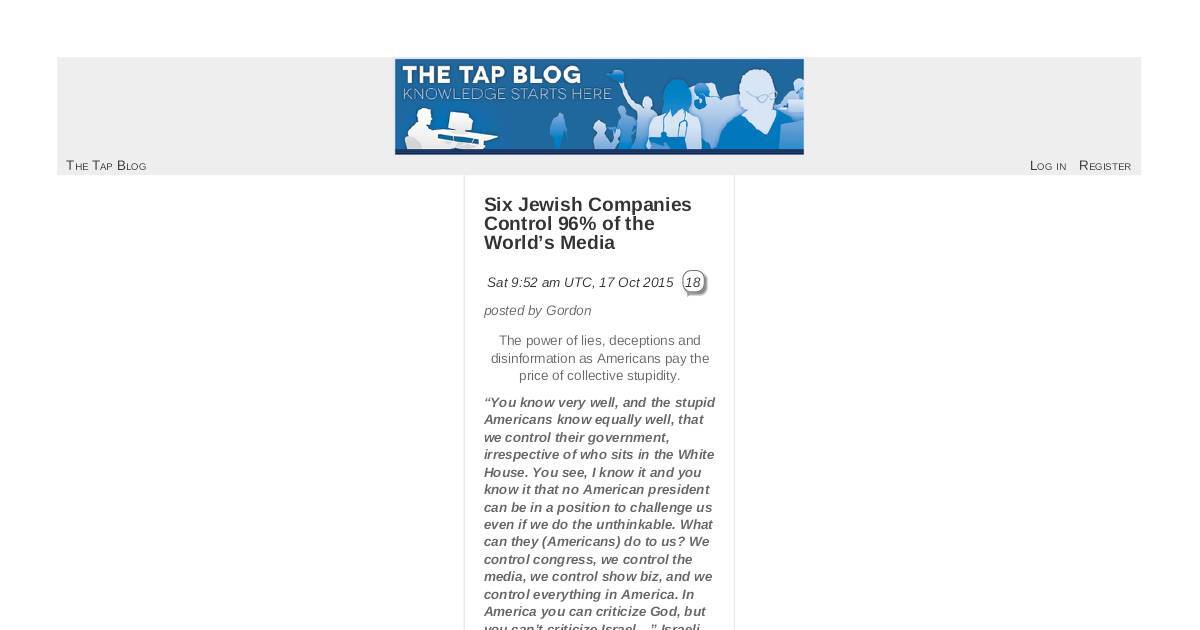Caption: 

"Screenshot of an article from a webpage featuring a grey banner at the top with the text 'The TAP Blog.' To the right of the banner, options to 'Log in' and 'Register' are visible. A blue central banner within the grey one prominently displays 'The TAP Blog' in bold white letters, accompanied by the tagline, 'Knowledge starts here.' Below these banners, graphic images of people with minimal detail appear—white bodies with blue hair and clothing. The article headline, 'Six Jewish Companies Control 96% of the World's Media,' is bolded and positioned prominently. It was posted by 'Gordon' on Saturday, October 17, 2015, at 9:52 AM. Below the headline, a provocative subtext reads, 'The powers of lies, deception, and disinformation as Americans pay the price of collective stupidity.'"